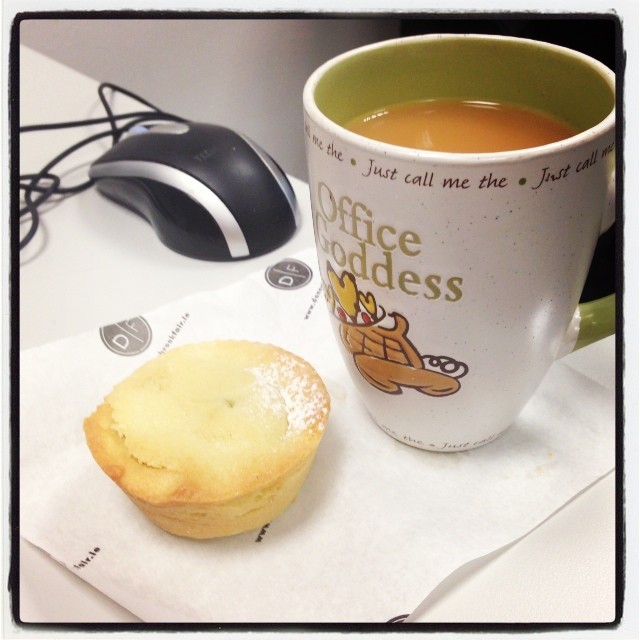This close-up image showcases a work desk featuring a white or cream-colored coffee mug adorned with green interior and handle. The mug prominently displays the phrase "Office Goddess" with the words "just call me the" repeated around its rim in a brownish color. Additionally, the mug's front includes an image with hearts and a telephone. The mug appears to contain coffee. It rests on a napkin next to a golden-brown muffin or piece of cake, dusted with powdered sugar. The napkin also bears some sort of emblem. Positioned off to the side, in the upper left quadrant, is a two-tone computer mouse with wires, combining shiny black and silver details. The table or desk underneath is white. This detailed scene portrays a cozy office moment.